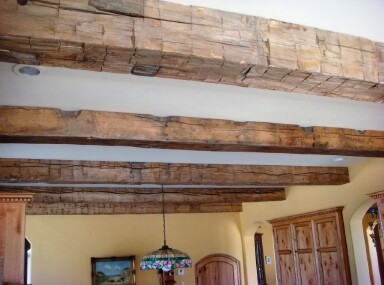Inside this room, an elaborate blend of rustic charm and vintage elegance captivates the eye. The ceiling, painted a soft white, is accentuated by five robust wooden beams, rugged and splintered, showcasing their age and authenticity. These beams extend in parallel lines, growing smaller with perspective, and contrast strikingly against the smooth ceiling. 

Suspended from one of these beams is a Tiffany-style stained glass chandelier, hanging prominently toward the left of center. Its vibrant composition features shades of yellow and pink with a distinctive green band encircling the center, hinting at intricate floral patterns.

The walls, painted a light yellow, host wooden elements that echo the ceiling beams' warm brown, weathered tones. On the left, partially obscured, hangs a landscape painting with visible rich details, adding artistic depth to the scene. Further examining the room reveals heavy wooden furniture, akin to armoires, whose craftsmanship parallels the aged beams above.

On the right side of the image, two arched structures hint at doorways or windows, both framed in matching wood, enhancing the room's overall cohesive aesthetic. A recessed light embedded near the top left corner adds a modern touch to the otherwise vintage interior. This room masterfully intertwines the old and the new, transporting one to a space where history and elegance coexist harmoniously.